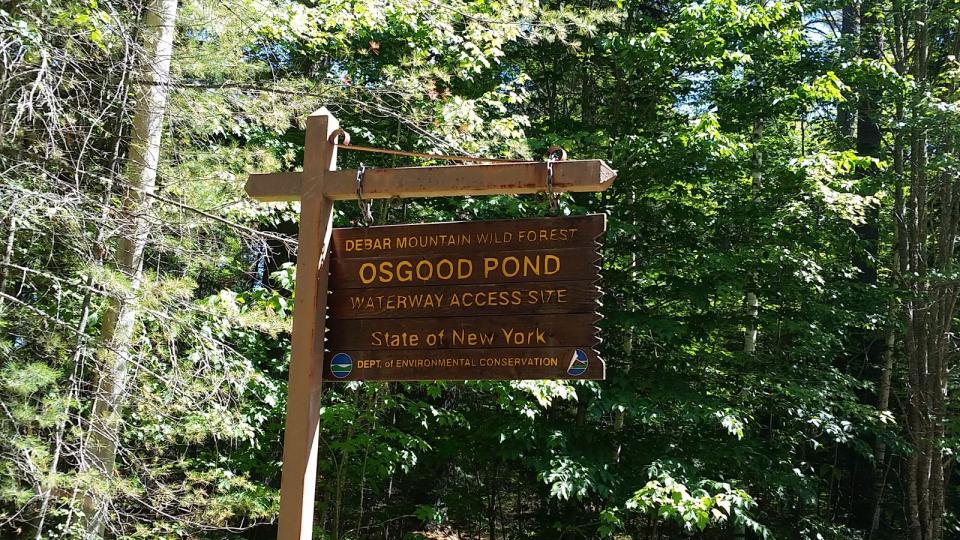The photograph captures a detailed scene in the outdoors, focusing primarily on a weathered wooden trail sign posted in a dense forest setting. The sign, which is made up of brown strips of wood, hangs from a horizontal beam attached with two chains to a vertical post. The text on the sign, written in yellow, reads from top to bottom: "Debar Mountain Wild Forest, Osgoode Pond, Waterway Access Site, State of New York, Department of Environmental Conservation." On either side of the phrase "Department of Environmental Conservation," there are two small, circular artistic renderings of mountains. The background features a bright sun illuminating a mix of barren branches and lush green foliage, creating a stark contrast between the sign’s aged appearance and the vitality of the surrounding forest, composed of tall evergreen trees and dense shrubbery. The natural, earthy tones of the scene give it a serene and rustic ambiance, indicative of a well-trodden wilderness path.